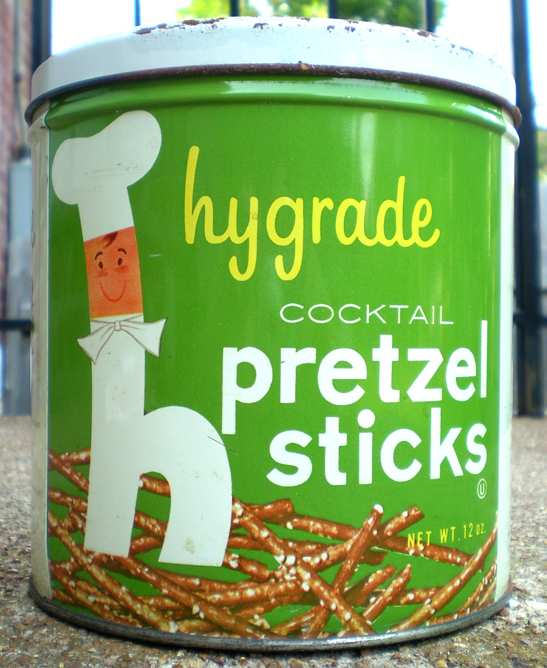This image features a large, lime green tin can labeled "High Grade Cocktail Pretzel Sticks." The can is adorned with an illustration of a pretzel character dressed as a chef, complete with hair-like bangs and a white bow tie. The pretzel character's body is cleverly shaped like an "H." The lower portion of the can displays multiple images of the pretzel sticks, with the words "Cocktail Pretzel Sticks" written in white. The can is topped with a white lid that appears significantly damaged, featuring numerous dents and chips. It is placed on a concrete pavement outdoors, with a house, an electrical box, and several blue poles visible in the background, adding context to the scene.